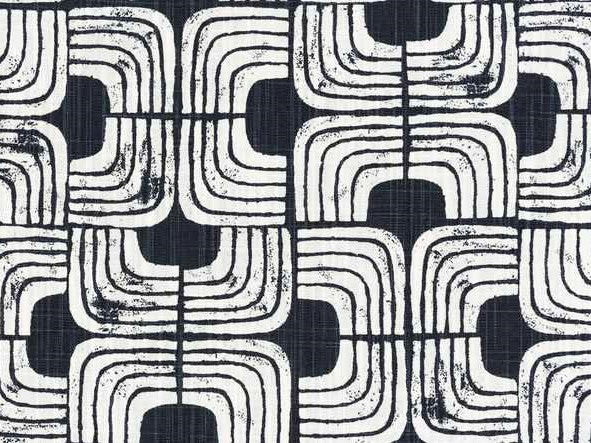This artwork is a rectangular image featuring a repeating tiled pattern with intricate geometric designs. The tiles consist of curved "L" shapes forming larger shapes that stack and interlock within a square format. Each of these composite tiles includes four right angles with rounded corners, resembling the shapes of capital "U" or lowercase "n." These tiles are rotated 90 degrees and mirrored across the image, creating a seamless pattern that runs both horizontally and vertically, covering the entire artwork.

The dominant colors are white and a deep navy blue or black. The white lines of the pattern are exceptionally thin, almost like scratch marks, forming a very fine plaid underneath the main design. This plaid is so delicate that it appears woven into the background, adding texture and depth.

Each "L" shape is segmented by five white lines separated by blue spaces, enhancing the visual complexity. The background of the pattern maintains the same dark hue with an underlying plaid, accentuating the white lines of the shapes. The overall effect is a balanced, rhythmic composition that is both visually striking and meticulously detailed.